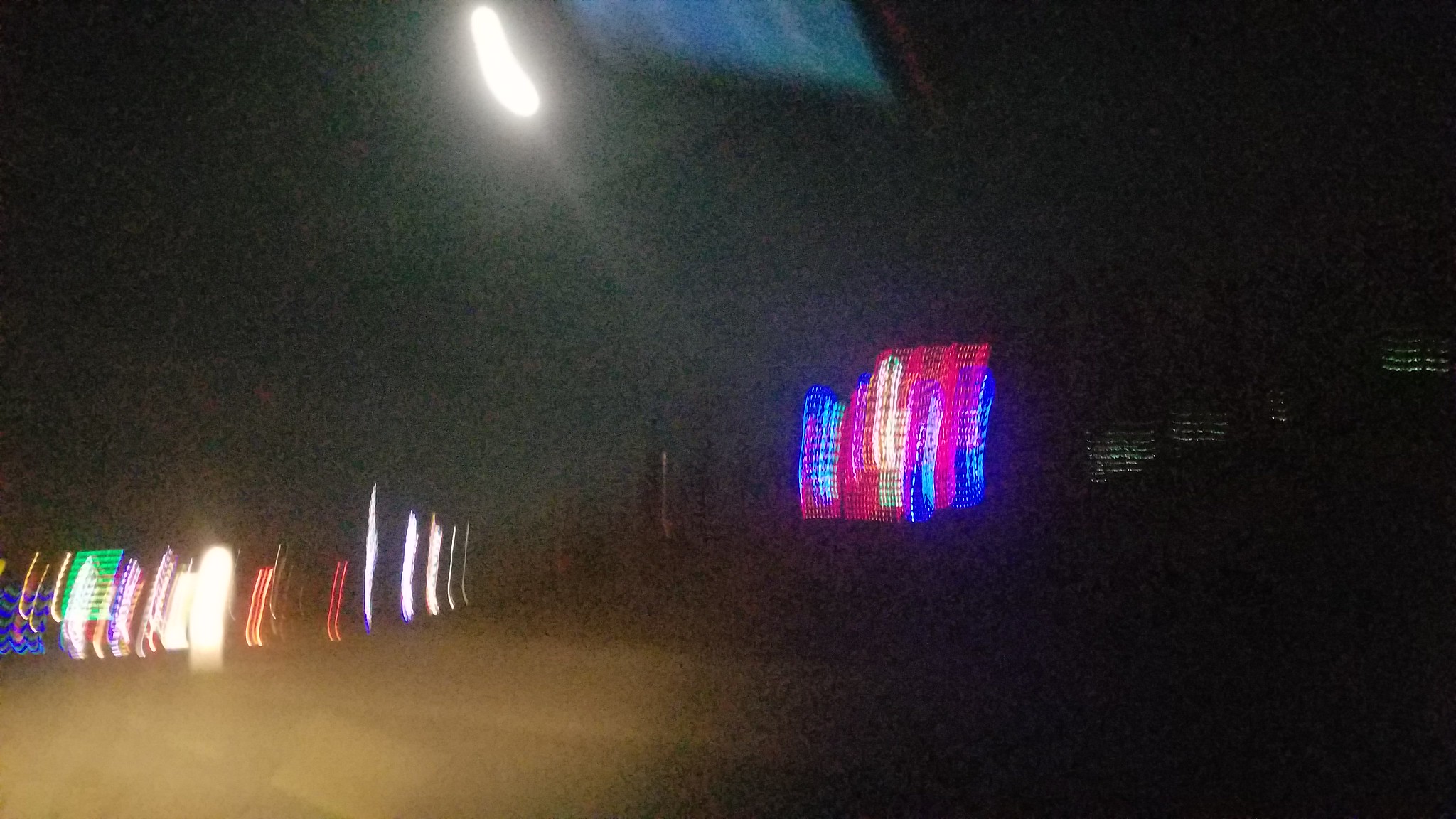This is a rectangular, horizontal color photograph taken at night, characterized by its significant blurriness and graininess. The primary elements are various lights scattered across the image, which dominate the composition and create a hazy, indistinct atmosphere. At the top of the photograph, there's an oval light that could be a streetlight, casting a haze over the scene. Adjacent to this light and partially cut off by the edge of the image is a rectangular shape, whose purpose remains unclear.

In the middle section of the photograph, a cluster of vertical lights in red, white, and blue emerges, suggesting the effect of capturing a moving object or the camera shaking. These vertical lines add to the sense of motion. Further down the slope, more vertical lights in an array of colors—white, red, purple, green—appear but are scattered more sparsely as they approach the edges of the image. On the left side, possibly against a building, there are additional lights in orange, blue, and green, which extend the colorful array but maintain the blurry and indistinct quality. Towards the right side and in the distance, very faint lights can be seen, though their exact details are obscured by the overall dim and blurry nature of the photograph.

The bottom left of the photograph suggests the presence of headlights, hinting that the photo might have been taken from a moving vehicle. This area includes various vertical white lines and hints of colors such as yellow and red, contributing to the chaotic and dynamic feel of the scene. The combination of hazy lighting and blurred forms creates an intriguing, though puzzling, nocturnal landscape.